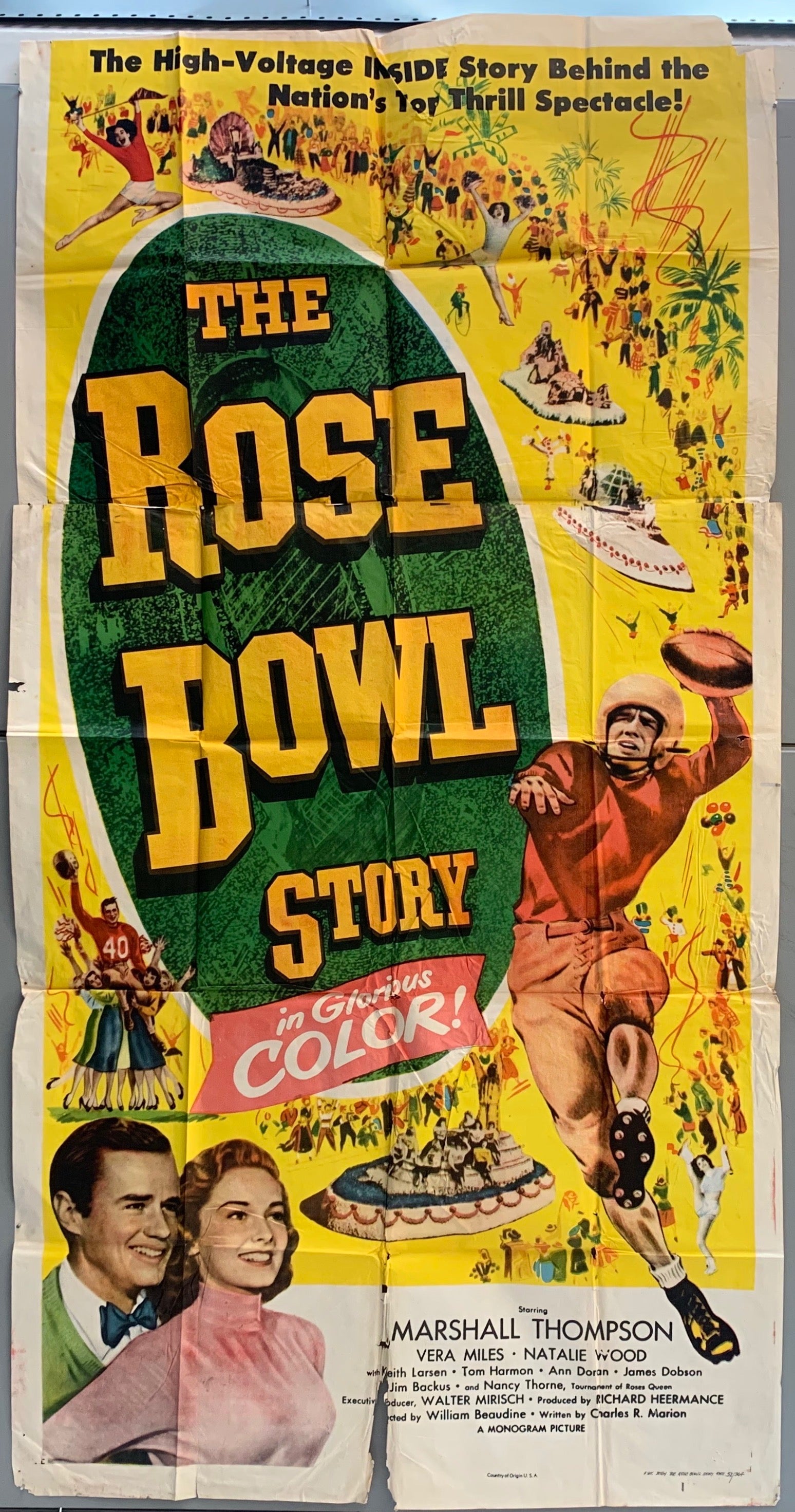The image is a vintage promotional poster for "The Rose Bowl Story." At the top of the poster, in bold black font, the headline reads, "The high voltage inside story behind the nation's top thrill spectacle." The central focus features the title "The Rose Bowl Story" in orange letters set within a green ellipse with a white border. 

The background of the poster is yellow with a white border, adding an aged, nostalgic feel. Surrounding the main title are small illustrations, including scenes of people playing sports and spectators watching. Notably, on the bottom right, there is a depiction of a rugby player in a red shirt and shorts, holding a ball in his left hand. Towards the bottom and slightly towards the left side, there is an image of a man and a woman; the man wears a white shirt, green jacket, and blue bow tie, while the woman dons a pink dress.

On the lower part of the poster, written on a pink ribbon in white letters, it says, "Starring Marshall Thompson, Vera Miles, Natalie Wood, with Keith Larson, Tom Harmon, Ann Doran, James Dobson, Jim Backus, and Nancy Thorne, Tournament of Roses Queen." Further below, it lists the creative team: "Executive Producer: Walter Mirisch, Produced by Richard Heermance, Directed by William Beaudine, Written by Charles R. Marion." Finally, at the very bottom, it declares, "A Monogram Picture."